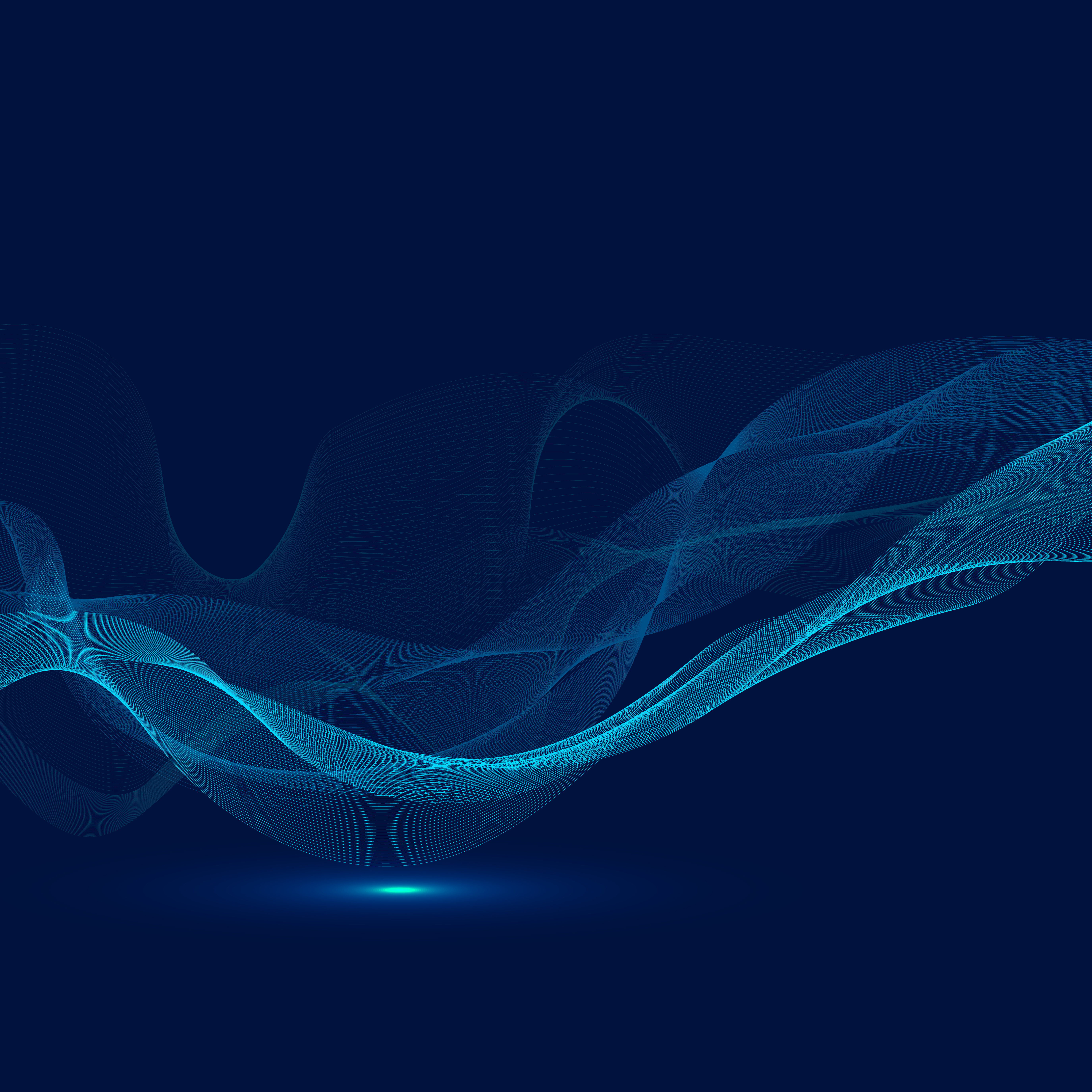The image depicts a computer-generated abstract pattern against a solid dark blue background, evoking the nostalgic feel of older-style screensavers. A series of wavy, smoky forms—ranging in color from light blue to light green—traverse the image from the middle of the left-hand side to the middle of the right-hand side. These waves undulate up and down, creating a sense of depth as some appear closer and others farther away. Most notably, towards the bottom center, a wave dips closest to an unseen ground, causing a bright, almost whitish-blue light to illuminate the area before quickly fading out. This light is particularly striking against the plain backdrop, adding a dynamic focal point to the image. The overall design is clean and clear, with no additional text or numbers to distract from the visual flow.